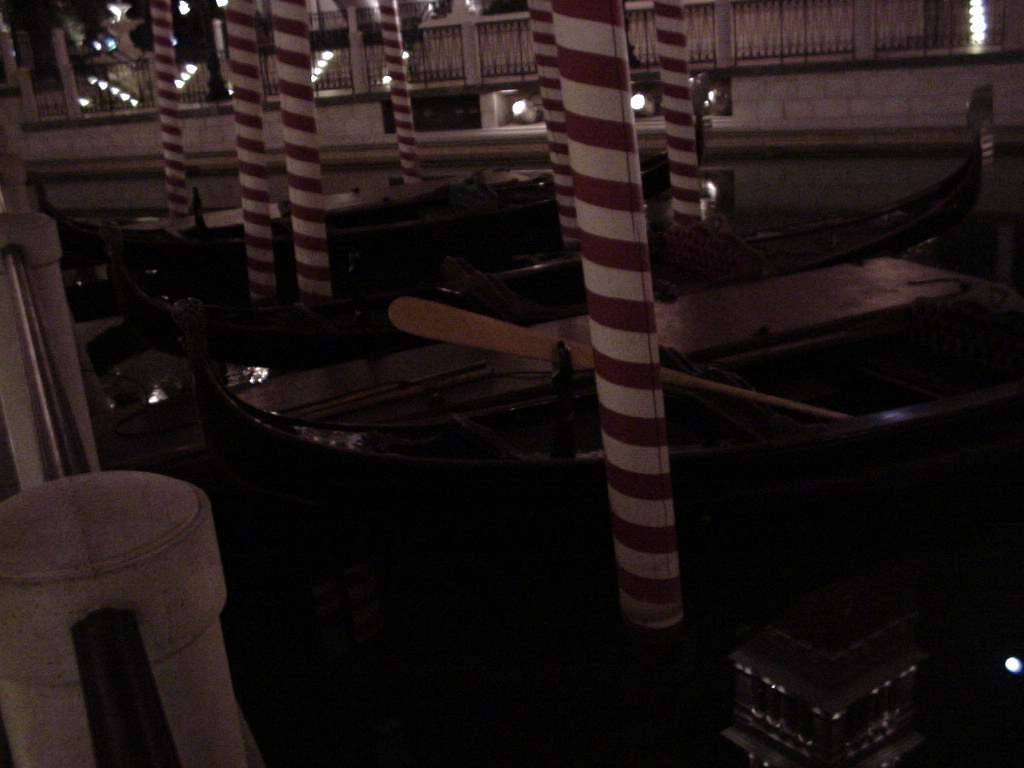In this dimly lit, nighttime outdoor scene resembling Venice, several brown wooden gondolas are docked in a dark canal. The canal is lined with numerous thick cylindrical poles, adorned with spiraling red and white stripes reminiscent of candy canes or barber poles. One gondola has an oar visible along its side. In the background, a white or light gray brick wall with black railings runs along the top, adorned with intermittent lights that cast a soft glow. To the left, there's a similar railing that appears to act as a handrail. The water and the sky both appear nearly black due to the low light, with multiple lights faintly illuminating the scene from different angles.